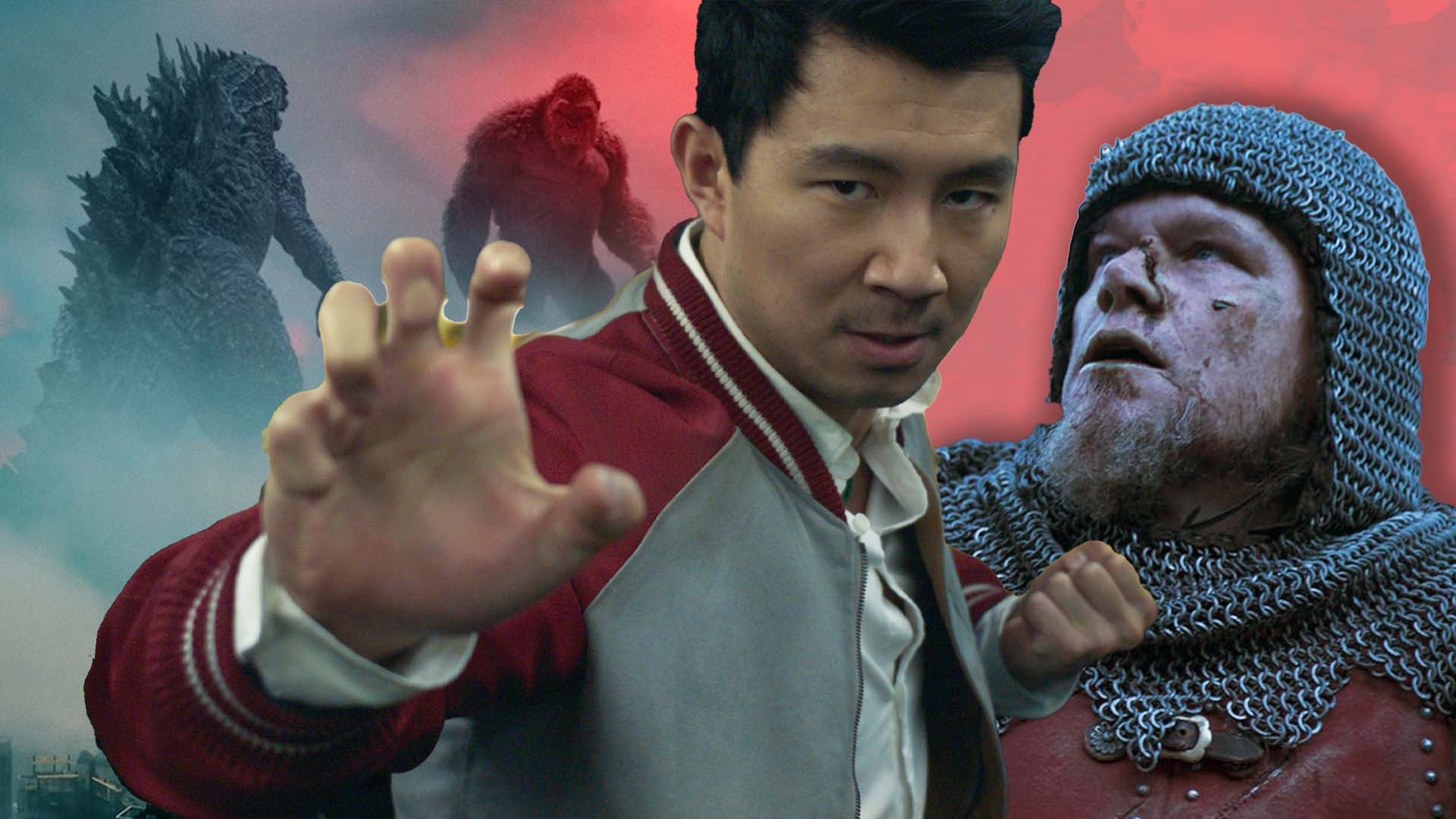The image is a captivating mashup of various movie characters set against a blurred pinkish-red and greenish-blue background. At its focal point is a young Oriental man in a Kung Fu pose, wearing a gray and magenta athletic jacket over a white button-up shirt. His intense brown eyes and claw-like hand reaching towards the camera add a modern, menacing touch. To his right stands a battle-worn knight, adorned in chain mail around his head and shoulders, with a cut down his nose, partially obscured by shadow. On the left, two iconic monsters are poised to clash: a vivid red King Kong and a brilliant blue Godzilla, their aggressive stances and scaly textures contrasting sharply. The overall composition gives the scene an intense, dynamic energy, as if blending scenes from different action movies into one dramatic poster.